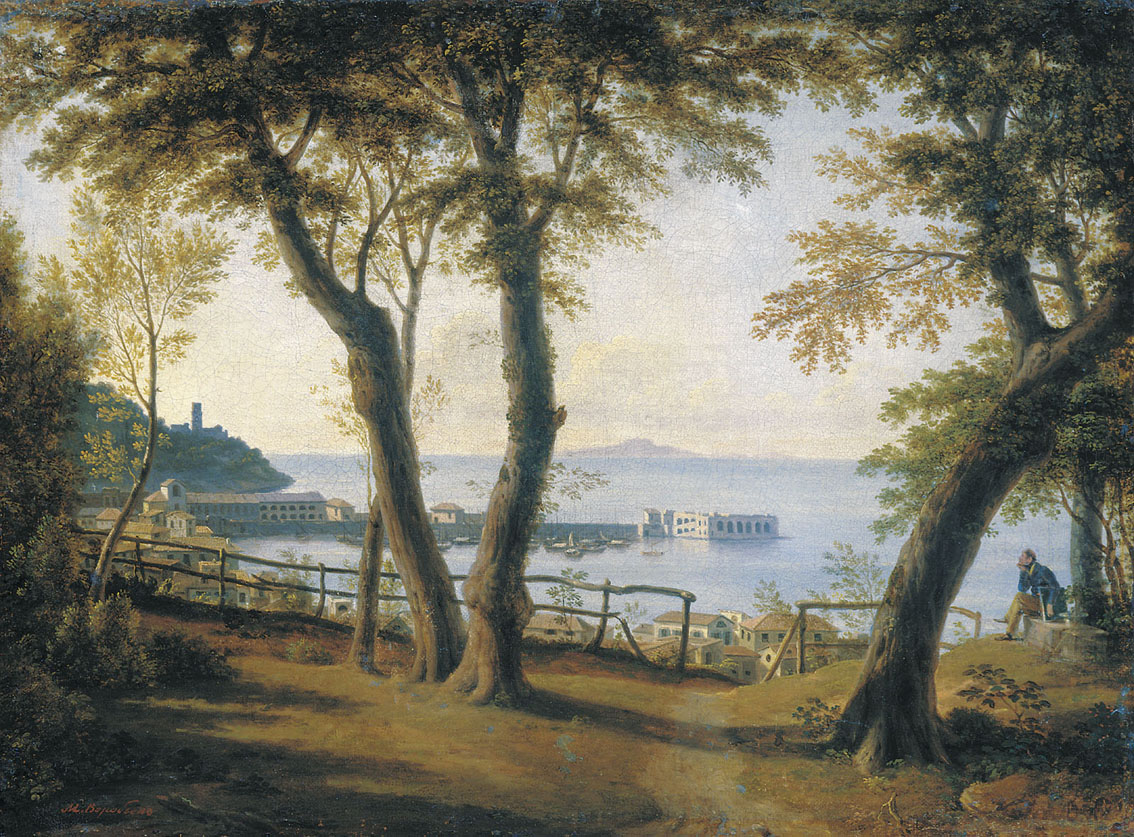The painting depicts a serene, picturesque lakeside or seaside landscape, with a clear, dominant horizon showcasing a blend of sky, water, and land. Central to the image is a quaint European-style town with distinctive buildings jutting into the water, their architecture suggesting an old-world charm. In the foreground, a small park-like setting with several trees encircles a worn, crumbling wooden fence, which extends across the width of the scene. The foliage, in autumn hues, adds a subdued vibrancy to the overall composition, evoking a sense of a sunny, yet calm fall day.

To the right of the painting, a gentleman dressed in 19th-century attire sits cross-legged on a stone bench, striking a contemplative pose with his right hand supporting his chin. He appears to be lost in thought, his gaze wistfully directed towards the scenic vista ahead. Beside him rests an ambiguous object that could either be a bag or a painting.

Beyond the fence lies the charming town, where buildings cluster near the water, and a pier stretches out, invitingly, into the sea. The left part of the painting features rolling hills and additional buildings, set against a shimmering body of water that extends toward distant landmasses on the horizon. The color palette of the artwork is an elegant mix of browns, beiges, greens, light blues, grays, blacks, and whites, capturing the tranquil essence of the landscape.